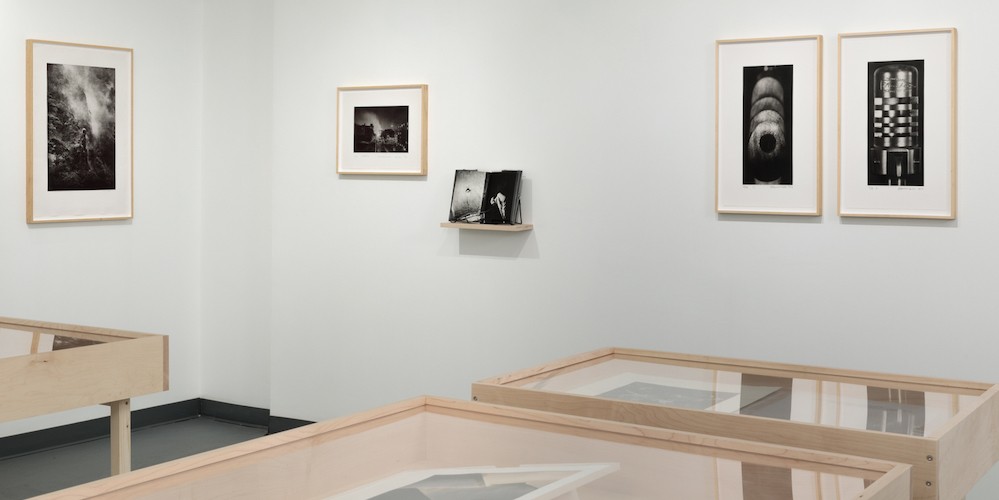This image depicts an art gallery or museum room with light blue walls adorned with black and white photographs. The wall trim is dark blue and the floor is gray. On the left side of the wall, there's a photograph framed in light brown wood, accompanied below by a glass-topped table of matching wood, showing one leg visible on the right. To the right of this setup, there are multiple light brown wood tables with glass tops, each enclosing additional black and white photographs. On the wall above these tables, four more black and white photographs are displayed, framed in light brown wood, with each frame featuring a white border around the photo. Additionally, a small built-in shelf holds more photos. The room’s design balances the light blue walls with the light brown wooden elements and black and white artwork, creating a serene and polished atmosphere suitable for an art exhibition.